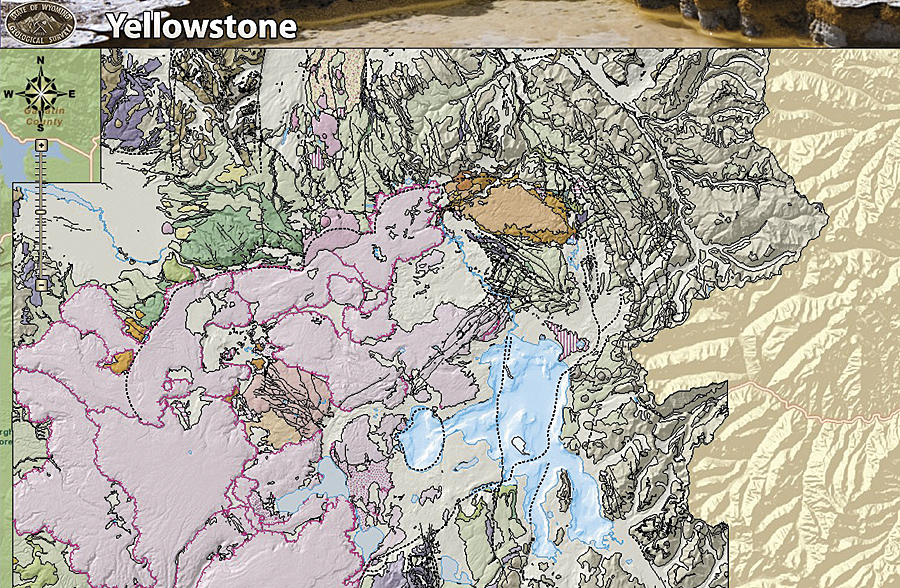This is an image of a detailed, colorful map of Yellowstone National Park from the State of Wyoming Geological Survey, with an emphasis on various geographic features distinguished by different colors. The title "Yellowstone" appears prominently in white text at the top left corner. To the left of the title, there's a stamp or emblem that depicts a mountain peak along with the words "State of Wyoming Geological Survey," although "Geological" is misspelled as "GIOlogical."

The map itself is rich in detail and color-coded: blue areas signify water bodies, mostly centralized, with light blue hues representing lakes and rivers. The eastern part of the map is predominantly beige, indicating mountainous terrain. Western regions are more colorful, with shades of pink, green, and gray, perhaps indicating different land types or park features. A mini-map appears in the upper left corner, featuring a small compass rose pointing north, south, east, and west, highlighted by a black and gold outline. This mini-map shows green denoting forested areas, blue for water, and a yellow-brown line indicating a road.

Black lines outline the different features on the map, with black dots likely representing roads. The map overall lacks a legend but includes these distinct color patterns—black jagged lines delineate the varied topography. At the top of the image, there's a real photograph of a dirt road bordered by green grass and gray rocks with moss, enhancing the map’s context within natural settings.